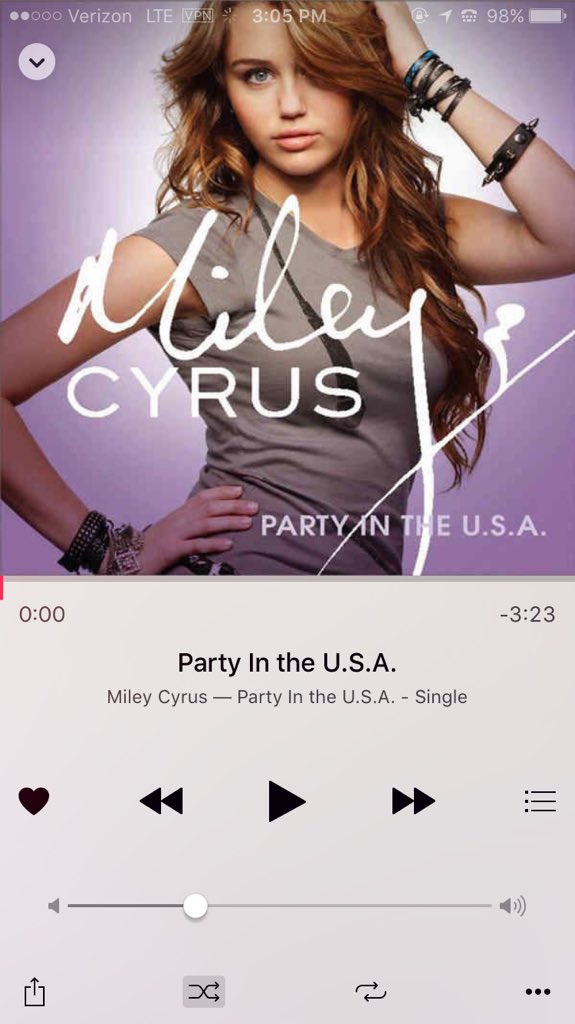This screenshot, taken from a smartphone locked screen, captures several details. The phone, serviced by Verizon, displays two bars of signal strength and LTE connectivity with an active VPN. The time reads 3:05 PM, and the battery is at 98%. Location services are enabled. The highlight of the screenshot is the music player interface showcasing Miley Cyrus's "Party in the USA" from her single. The song, which is 3 minutes and 23 seconds long, has not yet started playing. The music player presents standard options including shuffle, like, backtrack, play, fast forward, and a context menu indicated by three dots on the right side. Additionally, the interface features an image of a young Miley Cyrus as a long-haired brunette adorned with spike bracelets. This detailed representation displays the user's current activity of listening to Miley Cyrus's popular track "Party in the USA."